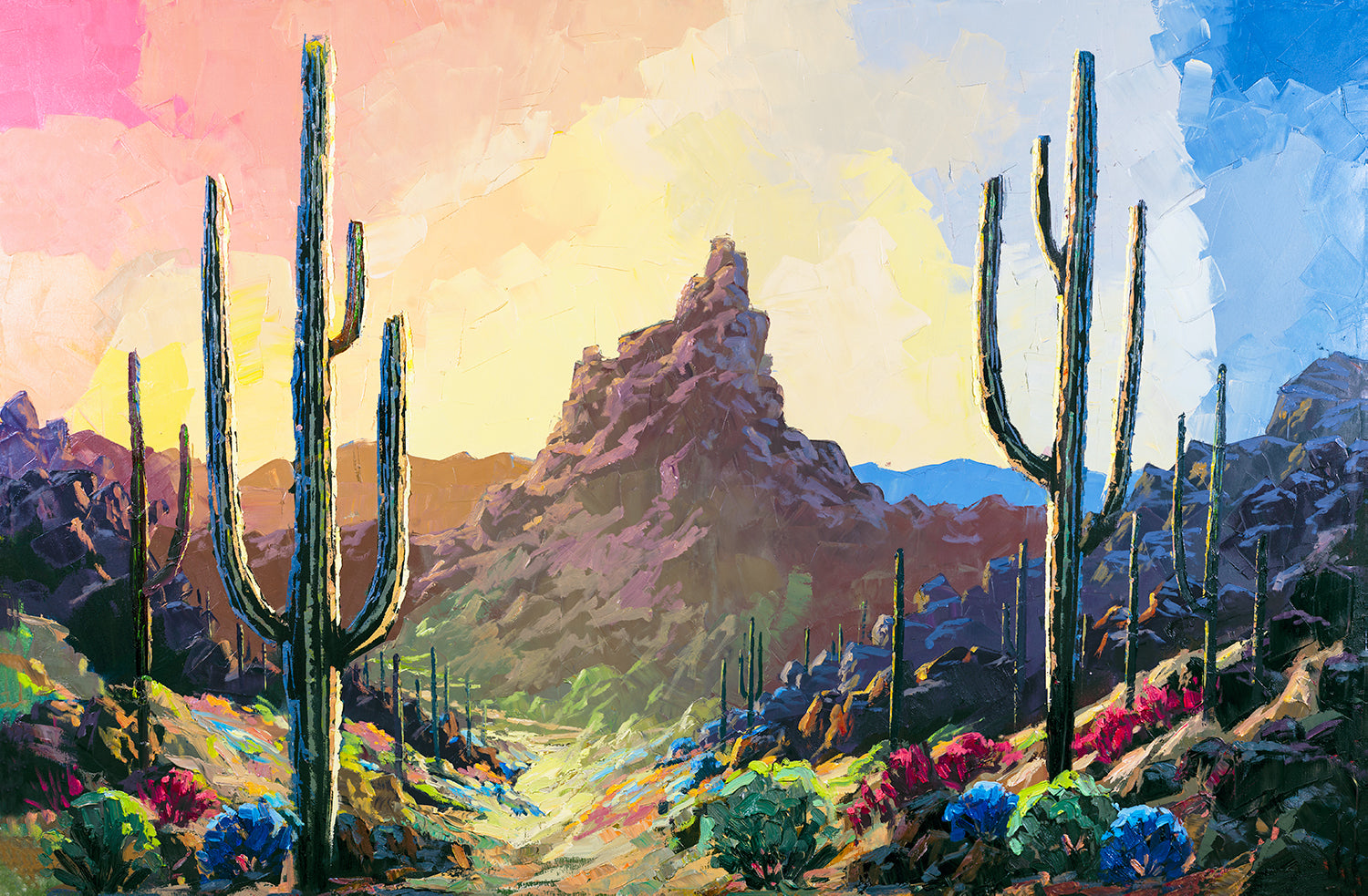The image is a vibrant digital painting of a desert scene, showcasing a landscape that almost resembles a computer graphic illustration. Dominating the center background is a tall, imposing rock formation composed of purplish and dark gray stone. To the right and left of this central feature are more mountain ranges, with those on the right appearing blue and those on the left displaying a mix of orange and brown hues.

In the foreground, typical saguaro cacti, with their arms curved upwards, add a striking greenish-blue contrast against the sandy and rocky terrain dotted with colorful bushes and flowers. These bushes and flowers display an array of greens, blues, reds, pinks, and purples, adding to the vibrant tapestry of the scene.

The sky overhead is a spectacle of bright, fluffy clouds rendered in a watercolor style, featuring a spectrum of colors including light yellow, orange, dark pink, magenta, blues, and a darker blue. This colorful sky lends a dreamy, almost surreal quality to the painting, casting a gentle yellow glow on the cacti and the landscape below.